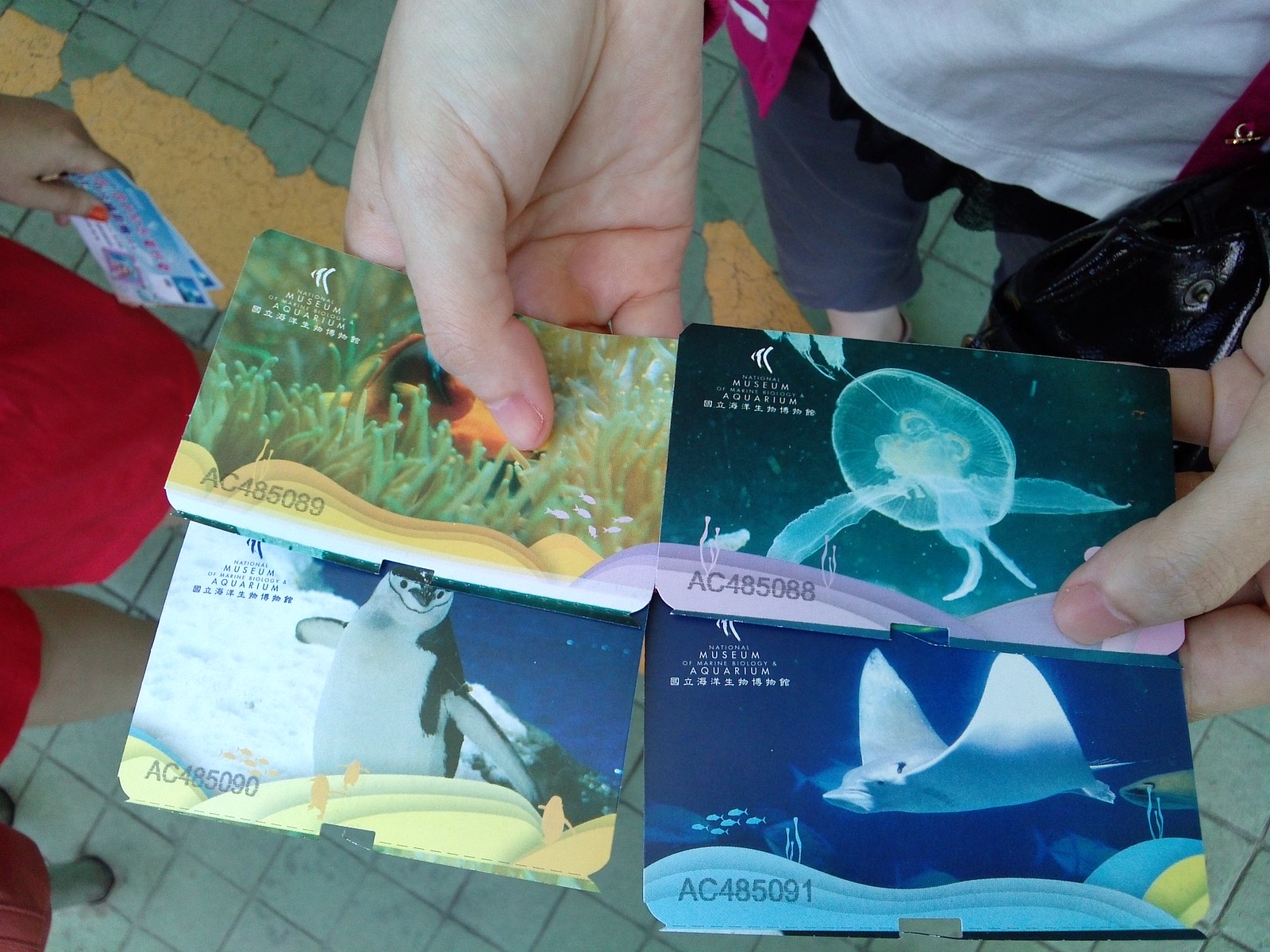In the image, we see two individuals showcasing what appear to be business card-sized magnets or entry cards, possibly as remembrances from visiting a museum and aquarium. The individual at the center, clad in a white t-shirt, red and grey trousers, and carrying a black bag, holds four cards. These cards prominently feature marine life: a jellyfish, a manta ray, a penguin, and a colorful fish swimming at the grassy bottom of the water. Each card is inscribed with the words "museum" and "aquarium," though some text is too small to decipher. Two hands, emerging from the top of the frame, also display two more cards, one in each hand. The cards, gripped by fingers adorned with orange nail polish, belong to a woman in a red shirt. Additionally, each card contains unique codes: AC485088, AC485091, AC485090, and AC485089. The background reveals a tile floor, adding a subtle contextual layer to the scene.